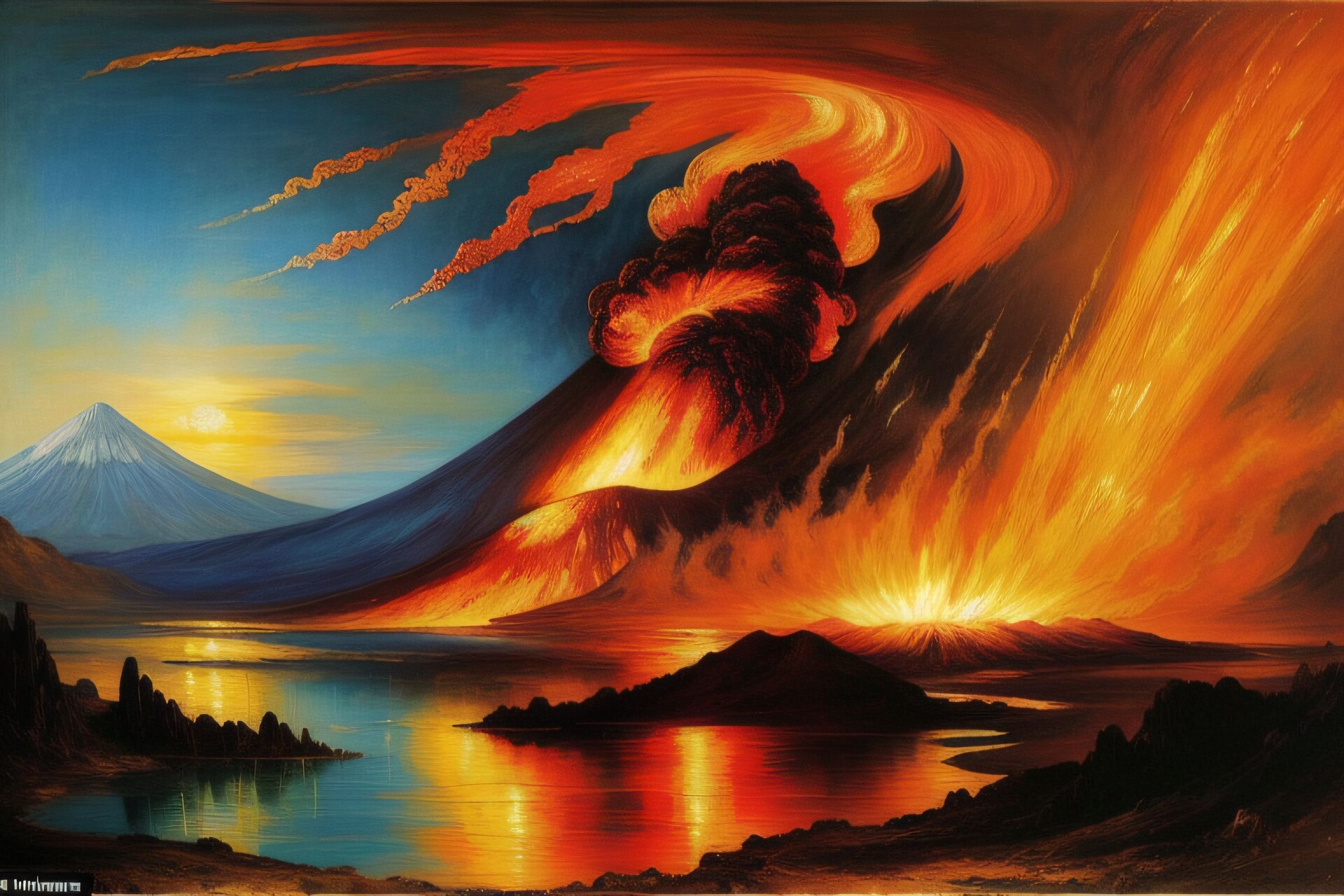The painting vividly captures a dramatic landscape divided into contrasting elements of tranquility and chaos. In the bottom third, rugged land and mountainous terrain extend into a vast body of water, reflecting the fiery spectacle above. On the right side of the image, a towering volcano is erupting, spewing vibrant red and orange flames and a plume of dark smoke high into the sky, casting an ominous presence. The eruption's intense colors—reds, oranges, and blacks—are mirrored in the water below. In stark contrast, the top left portion of the painting features a serene scene of bright blue skies with the sun gently peeking over a sharp, triangular mountain. This juxtaposition of the left’s peaceful, sunlit sky against the right's volatile eruption creates a compelling dynamic, symbolizing a battle between light and darkness, good and evil. The painting's overall clarity and vibrant colors further enhance the natural beauty and dramatic tension of the scene.